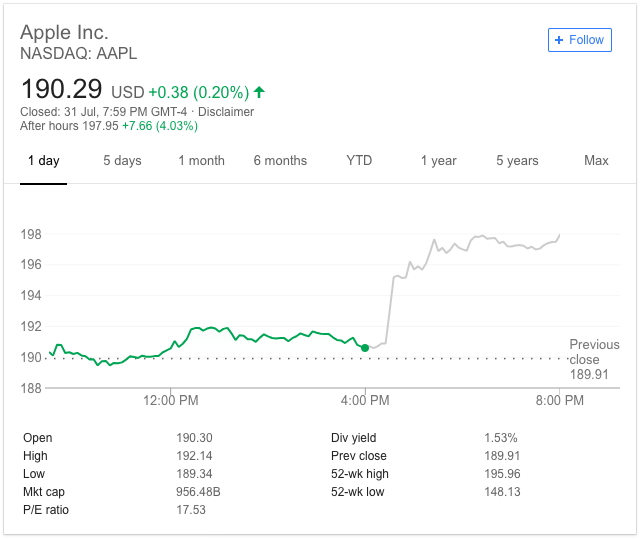This image is a screenshot from a financial website or app with a clean, white background. 

In the upper left corner, the heading "Apple IMC" appears in gray font. Directly below this, the text "NASDAQ: AAPL" is prominently displayed. In the upper right corner, there's a blue-outlined rectangle containing a plus sign and the word "Follow" in blue font.

Below the NASDAQ label, the stock price is shown as "190.29 USD," followed by a green arrow pointing upwards, indicating a positive change by "+0.38 (0.20%)." Beneath this information, a note reads "Closed 31 July 7:59 p.m. GMT," with a disclaimer mentioning after-hours trading data: "197.95 +7.66 (4.03%)."

Further down, a graph is presented, offering various timeframes for viewing: "1 Day," "5 Days," "1 Month," "6 Months," "Year to Date," "1 Year," "5 Years," and "Max." The graph itself features a black line, with the y-axis on the left side ranging from 198 to 188, and the x-axis at the bottom spanning from 12 p.m. to 8 p.m. The data indicates that the stock price began to rise notably after 4 p.m.